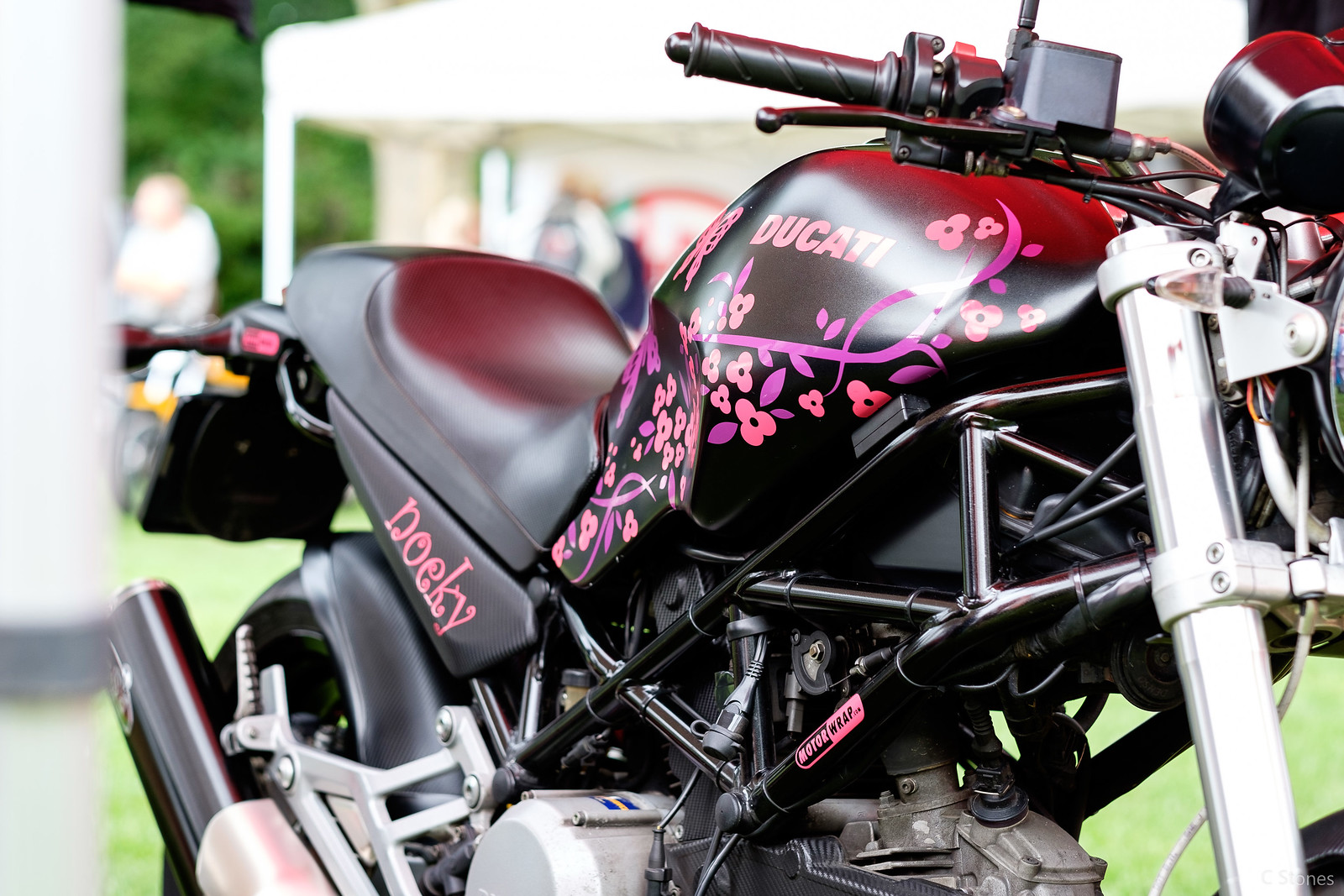The close-up horizontally aligned rectangular image captures the intricate details of a red and black Ducati motorcycle adorned with pink and purple floral designs. The word "Ducati" is prominently displayed on the side of the front, and "Naki" is printed on the side of the seat, suggesting it might be a personalized vehicle. The motorcycle's handlebars and brakes, matching in the reddish-black color scheme, are clearly visible. The background of the image is deliberately blurred, yet it reveals a man and some trees to the left, as well as a white post with a matching ceiling structure, hinting at an outdoor setting. Additionally, green grass is observable in the lower right-hand corner. The setting appears to be a public gathering, indicated by the presence of various people, bushes, and possibly another motorcycle in the backdrop. The overall image suggests a vibrant, daylit outdoor scene, focusing primarily on the artistically decorated motorcycle.